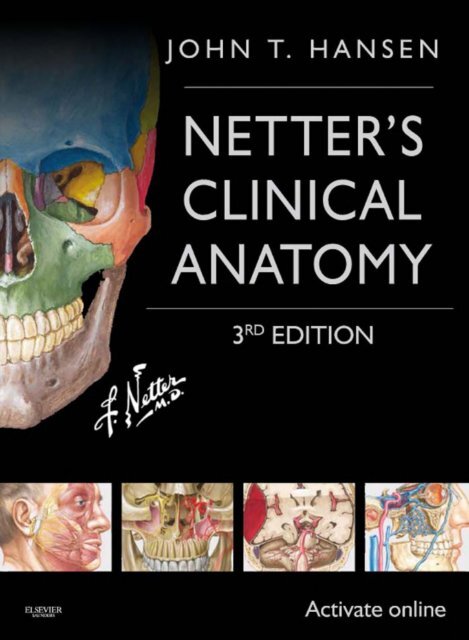The image is a vertical, rectangular book cover with a black background. It features the title "Netter's Clinical Anatomy, Third Edition" at the top in white letters, flanked by thin horizontal lines. The author, John T. Hansen, and the signature "J. Netter, MD" are also displayed. The cover shows a detailed illustration of the left half of a human skull, with different regions color-coded in blue, green, yellow, and tan, delineating various anatomical sections like the facial bones and orbital regions. Below the skull illustration, there is a strip of four smaller images depicting anatomical details: muscles of the face, possibly glands, a cross-section of the brain, and facial veins and arteries. The bottom right corner of the cover reads "Activate Online" in white font, and the publisher Elsevier is also noted.